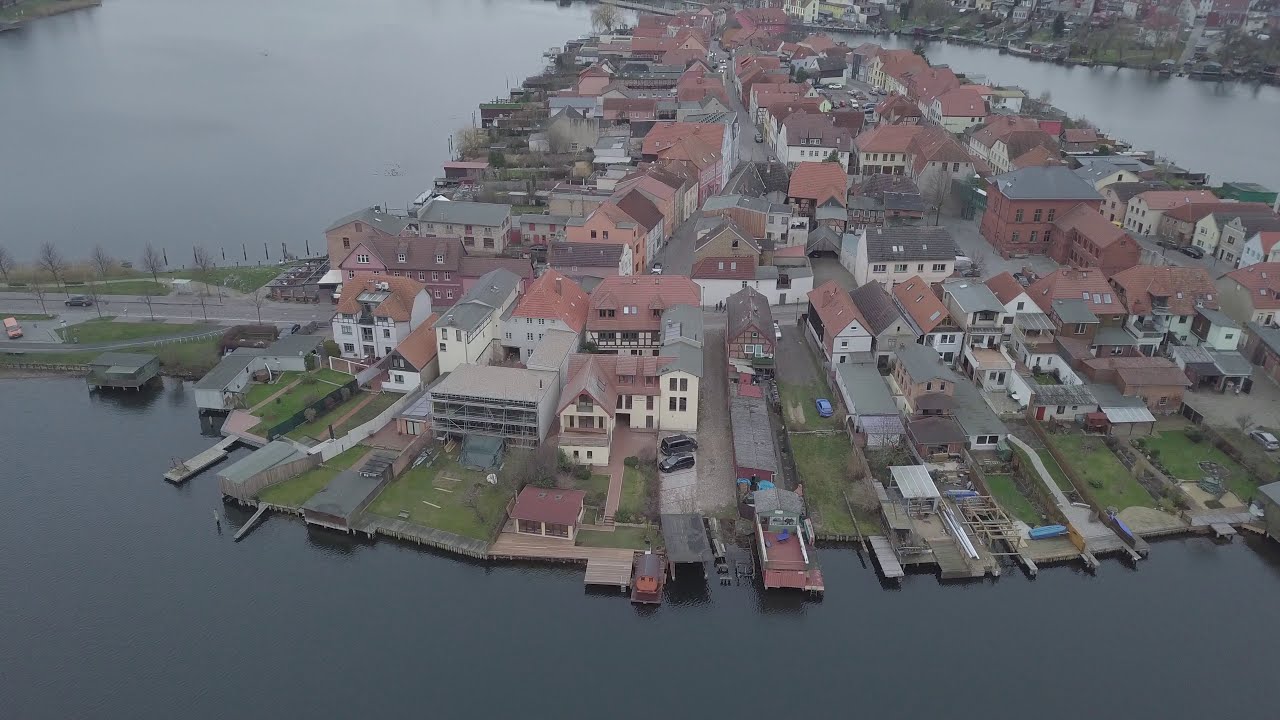This aerial photograph showcases an affluent, European-style community situated on a picturesque isthmus, surrounded by a serene body of water. The neighborhood is comprised predominantly of large, two to four-story brick houses with red roofs, embodying a charming architectural uniformity. The homes feature meticulously maintained grassy yards that gently slope towards individual docks, providing direct access to the waterway. Some homes have decks extending over the water, suggesting potential for recreational activities, although no boats are visible in the image. Prominent in the foreground are two grand homes flanking a smaller one, each with their own waterfront access. To the left of the smaller home is a paved area that appears to serve as a communal parking or possible boat slip area for non-residents. The layout behind these foreground homes reveals neatly arranged rows of similar structures, delineated by narrow roads. The image provides a sense of an exclusive enclave, almost entirely encircled by water, aside from what appears to be a three-lane road granting access to the mainland. The absence of a visible horizon emphasizes the expansive continuity of this idyllic waterside community.